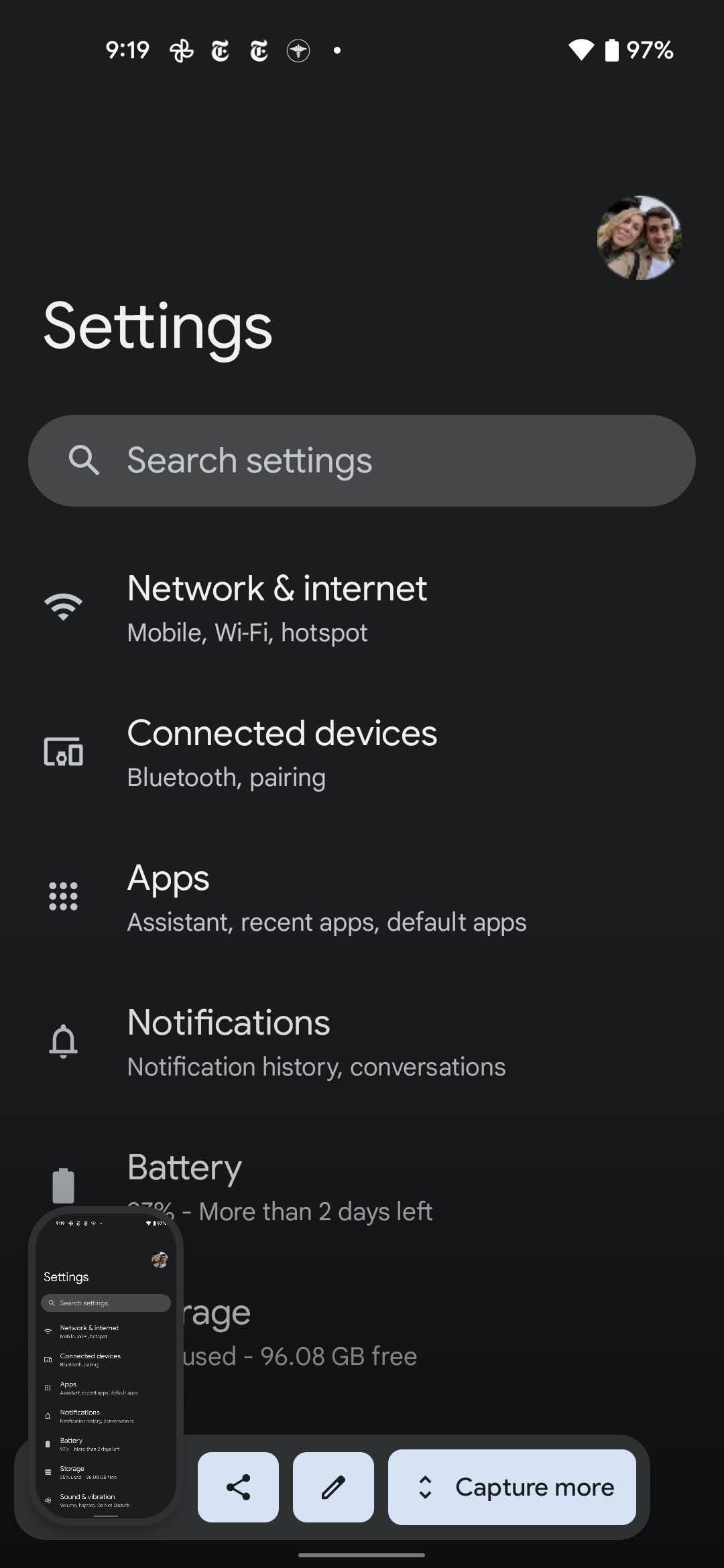This is a detailed screenshot of a smartphone's settings page. At the top of the screen, a status bar displays various icons in white, including those indicating battery level, current time, and background-running apps. Below this status bar, on the right side, there is a circular profile picture featuring a man and a woman with their heads close together. Directly beneath the profile picture, the word "Settings" is prominently displayed. 

A dark grey search bar is positioned below the settings title, allowing users to perform specific searches within the settings menu. Below the search bar, there is a categorized list of features, including "Network & Internet," "Connected devices," "Apps & notifications," "Battery," and "Storage." 

In the bottom left corner of the screenshot, there is a smaller, inset screenshot showing the same settings page, creating a "screenshot within a screenshot" effect.